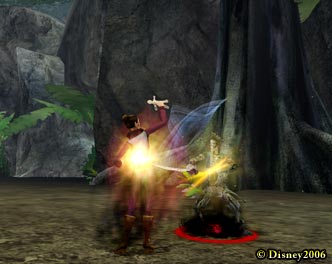This is a small, square image that appears to have been cropped or resized, creating a somewhat blurry and unclear appearance. In the bottom right corner, there is a distinctive yellow copyright symbol that reads "Disney 2006." The setting features a backdrop of gray and black stones, reminiscent of a cave or dark castle, with some green leaves peeking out on the left side and a large brown tree with exposed roots on the right. The ground below is a mix of brown, light tan, and black hues. In the center, two characters are depicted, seemingly engaged in a magical or combat scenario. The character on the right has a black and red ring beneath them, facing the character on the left, who is holding a luminous white light figure above their head. The scene is illuminated with vibrant flashes of yellow light, outlined in red, with streaks of blue, purple, and pink adding to the dynamic action.